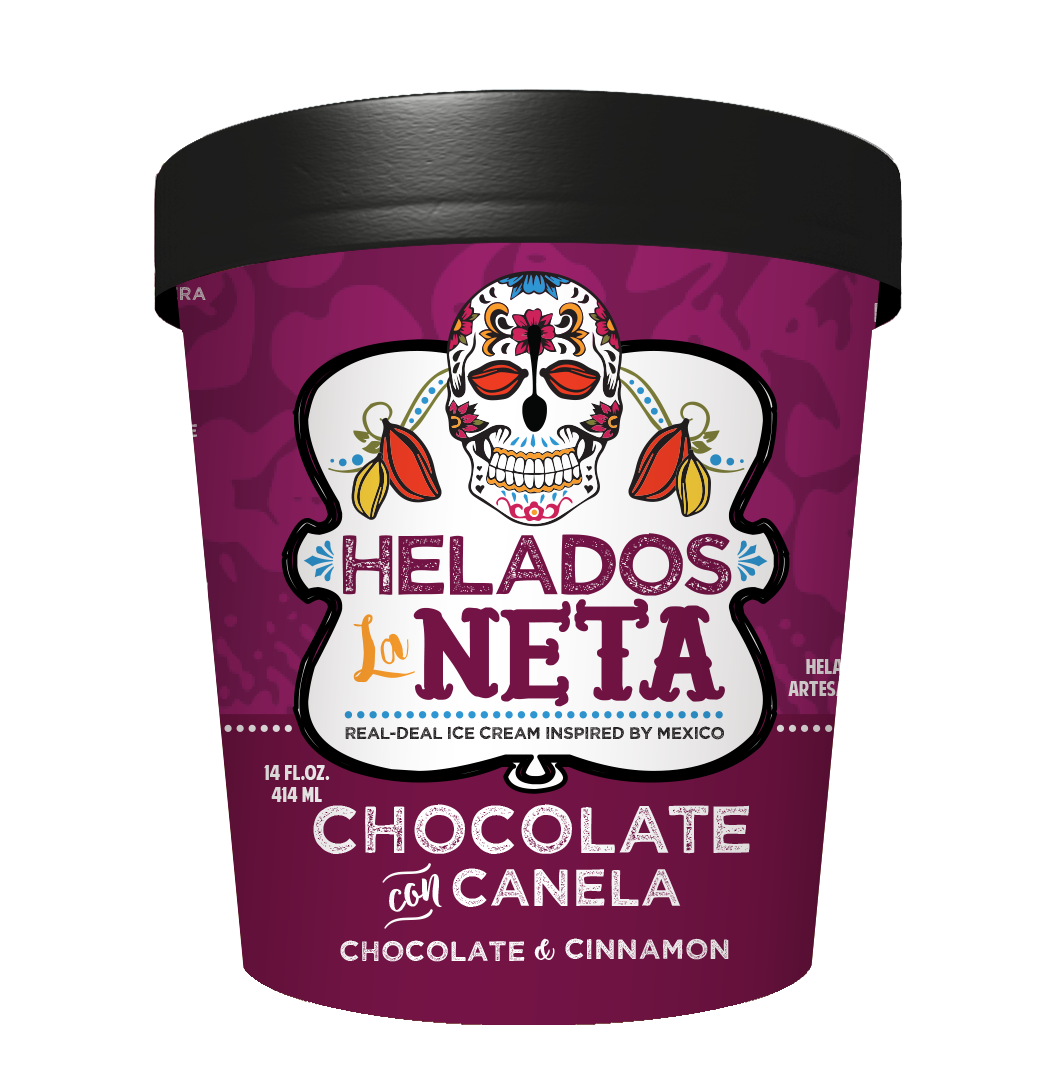The picture is a close-up of a 14-fluid ounce (414 milliliters) ice cream container from the brand Helados La Neta. The container tapers down slightly, resembling a pint-sized cylindrical bottle made of what looks like purple plastic. The label features a striking dark purple backdrop with a splash design in lighter purple hues. At the center, there is an ornate Day of the Dead skull with multicolored floral patterns, braids, and leaves. Above the skull, the text reads "Helados La Neta" within a white, pillow-shaped insignia. Below this, the label states "Real Deal Ice Cream, Inspired by Mexico" in smaller purple text. The flavor listed is "Chocolate con Canela," with the English translation "Chocolate and Cinnamon" beneath it. The container has a black lid and includes details about these features in white and purple writing.